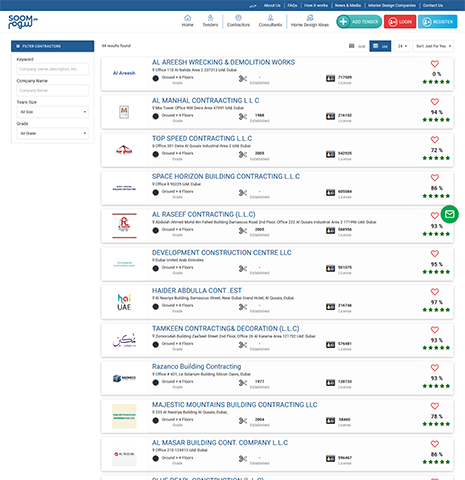Screenshot Description: Website Directory Page

At the top of the screenshot, there is a blue navigation bar with options reading "About Us," "FAQ," "How It Works," "Mobile," "Interior Design," and "Contact Us." Below this bar is the website logo, which spells out "SOOMROGW." Directly beneath the logo, there is a search bar where users can search by keyword, company name, and other options that are not entirely visible.

The main section of the page displays the text "94 results found," indicating the number of search results yielded. The results list companies involved in contracting and demolition work, including:
1. Al Arish Wrecking and Demolition Works
2. Al Manhall Contracting LLC
3. Top Speed Contracting LLC
4. Space Horizon Building Contracting LLC
5. Al Rasheed Contracting LLC
6. Development Construction Center LLC
7. Haider Abdullah Contractor EST
8. Tamkeen Contracting and Decoration LLC
9. Rosanco Building Contracting
10. Majestic Mountains Building Contracting LLC
11. Al Mazier Building Contractor Company, LLC